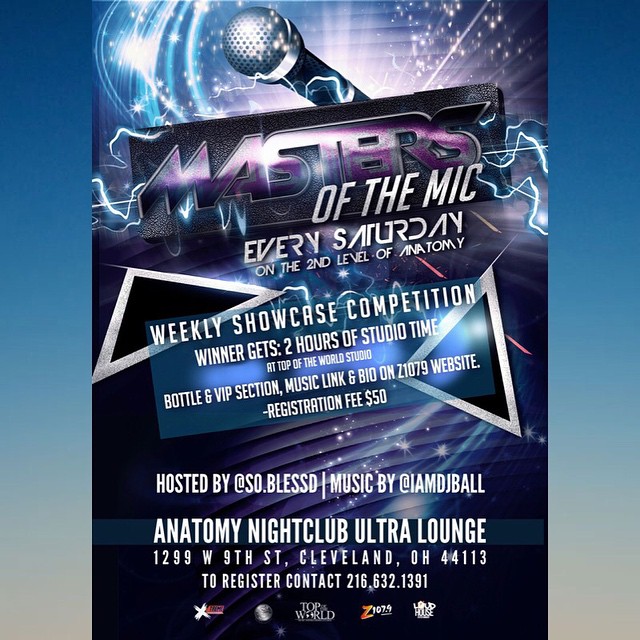This vibrant advertisement features a dynamic image of a microphone emitting lightning and sparkles, set against a gradient background that transitions from dark blue at the top to beige at the bottom. The flyer announces: "Masters of the Mic" in striking purple letters, with lightning accents. It promotes a weekly showcase competition held every Saturday on the second level of Anatomy Nightclub Ultra Lounge, located at 1299 West 9th Street, Cleveland, Ohio, 44113. The competition winner is awarded two hours of studio time at Top of the World Studio, along with a bottle and VIP section. More details and music links can be found on the Z107.9 website. The registration fee is $50, with the event being hosted by @soblest, and music provided by @iamdjball. For registration, contact 216-632-1391. The advertisement is adorned with a few logos of sponsors at the bottom, and a light blue border frames the left and right sides of the image, adding to the visual appeal.